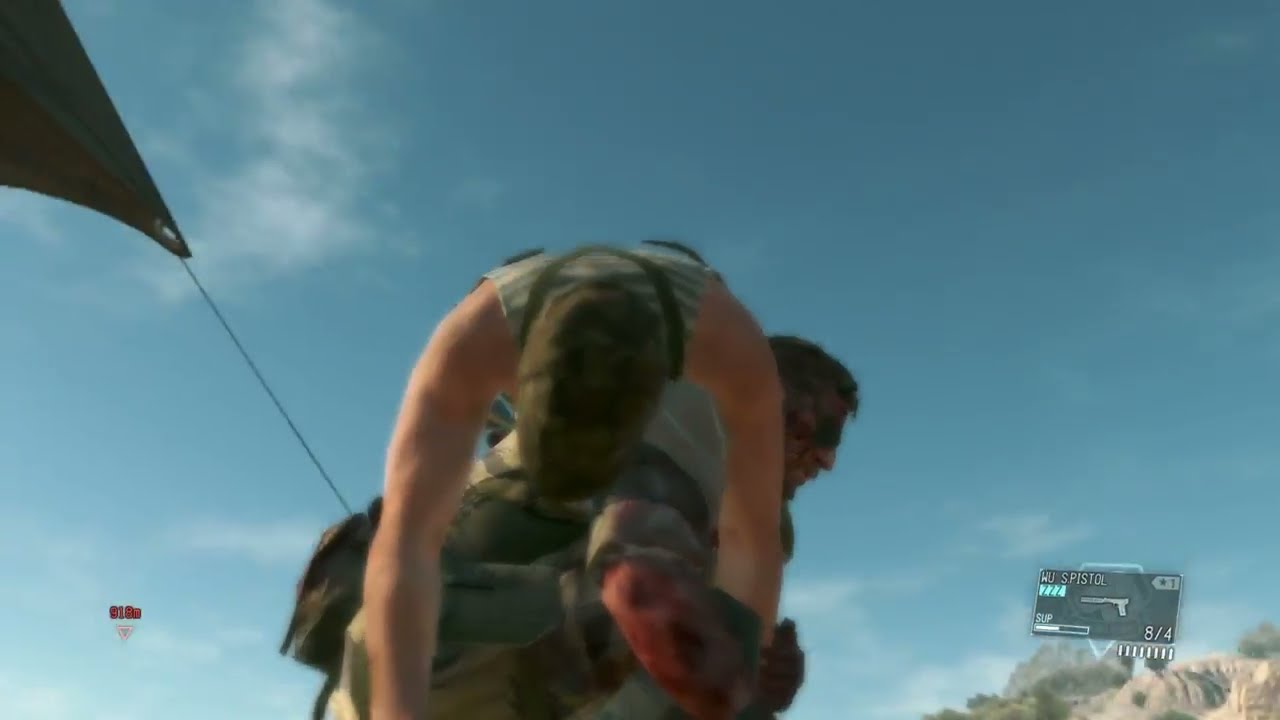This detailed screenshot from a video game depicts a kneeling character in the center, dressed in red clothing, with a long gun strapped to their back. The character is positioned on a patch of grass surrounded by green bushes. In the background, a couple of old, somewhat dilapidated houses with yellow walls and multiple doors, including boarded and colored ones, can be seen. Beyond the buildings, a distant brown, rocky hill with patches of trees is visible against a blue sky dotted with clouds. The game's interface is evident in the bottom right corner, displaying various icons and stats, including numbers and a label that reads "pistol," indicating the character's current weapon. The resemblance to classic video game graphics is notable, yet they maintain a middle-ground quality—not the most advanced, but sufficiently detailed for immersive gameplay. The setting seems desolate, with the crouching character appearing ready for a potential enemy ambush in a first-person shooter scenario.